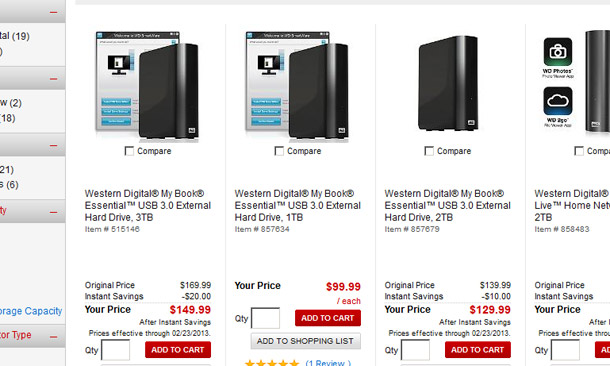The image depicts a web page featuring a product listing for the "Western Digital MyBook Essential USB 3.0 External Hard Drive 3TB." The left side of the web page is partially cropped, showing various filters represented by numbers in parentheses against a gray background. The right side features a clean, white background with a distinct gray line running horizontally at the top. Just below this line is an image displaying a computer system with a separate tower. 

Directly beneath the image, there is a checkbox labeled "Compare." Following this is the product title, "Western Digital MyBook Essential USB 3.0 External Hard Drive 3TB." The item is identified by a unique item number, #515146. The original price of the product is listed as $169.99. An "Instant Savings" discount of $20 is applied, reducing the price to $149.99. 

Below the price details, there is a field for entering the desired quantity of the item, adjacent to a large red "Add to Cart" button. The section is clearly organized, providing all necessary information for a potential buyer to make a purchase decision.